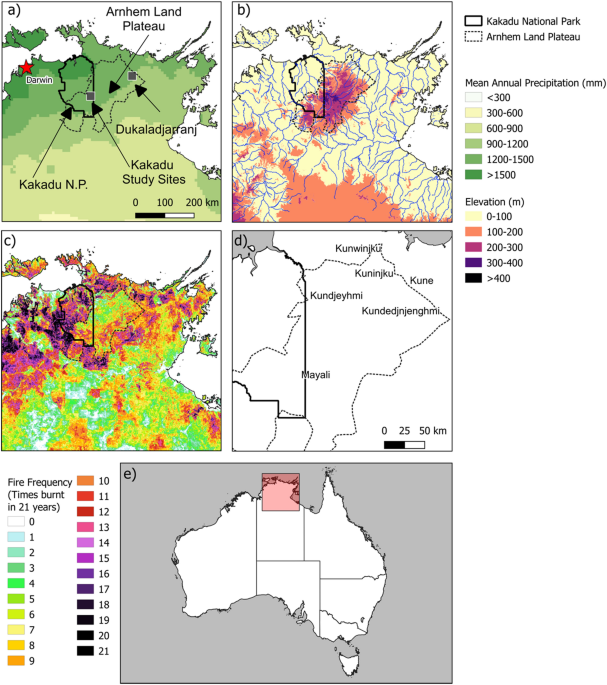The infographic consists of five maps labeled A, B, C, D, and E, each depicting fire frequency over the past 21 years in different regions of northern Australia. The top left map (A) highlights the Arnhem Land Plateau and Kakadu National Park, indicating a fire frequency of 2 to 5 fires per year, with Darwin as the nearest capital. Map B does not specify a region but shows a high fire frequency, particularly in one area experiencing up to 15 fires annually. Map C, also unnamed, reveals a concentrated area in the northwest corner with up to 21 fires annually, while most other areas have 3 to 10 fires per year. Map D, featuring regions such as Meali and Koonwipiju, shows no fire activity. The bottom map (E) provides a broader view of Australia with a red square focusing on the top middle portion, where the other maps are close-ups. The maps use various colors to represent fire frequency, mean annual precipitation, and elevation, with keys provided in the upper right and lower left portions of the infographic for reference.